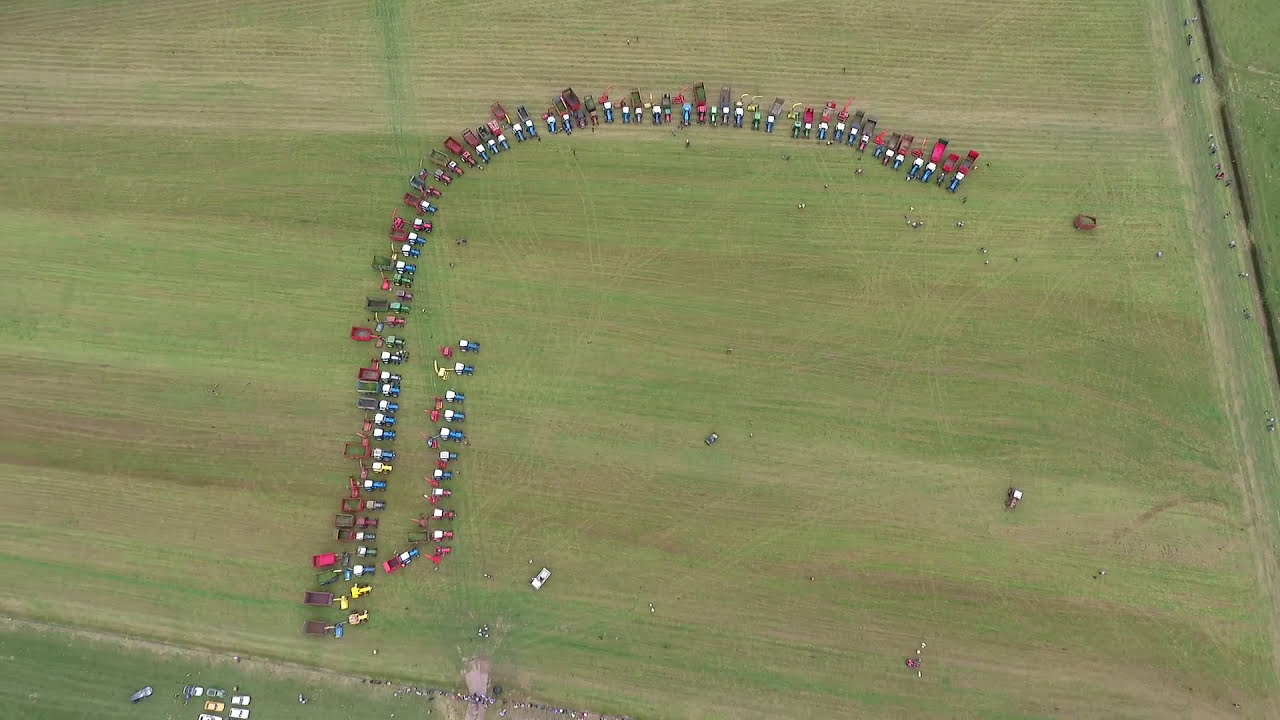The image showcases a vast, horizontal grass field captured from an aerial perspective. In the foreground, roughly ten vehicles, resembling pickup trucks or matchbox cars, are carefully arranged in a precise formation to create a distinct and elaborate design. The design, intricately composed of vibrant colors—red, blue, and white—sprawls across the grass. Additionally, nearby, there appear to be two lines of people or objects, adding more colorful elements including yellow, purple, blue, white, and pink. The first colorful line starts from the middle left, curves back, and then swings to the right, while the second, shorter line, begins slightly further back and extends straight without curving.